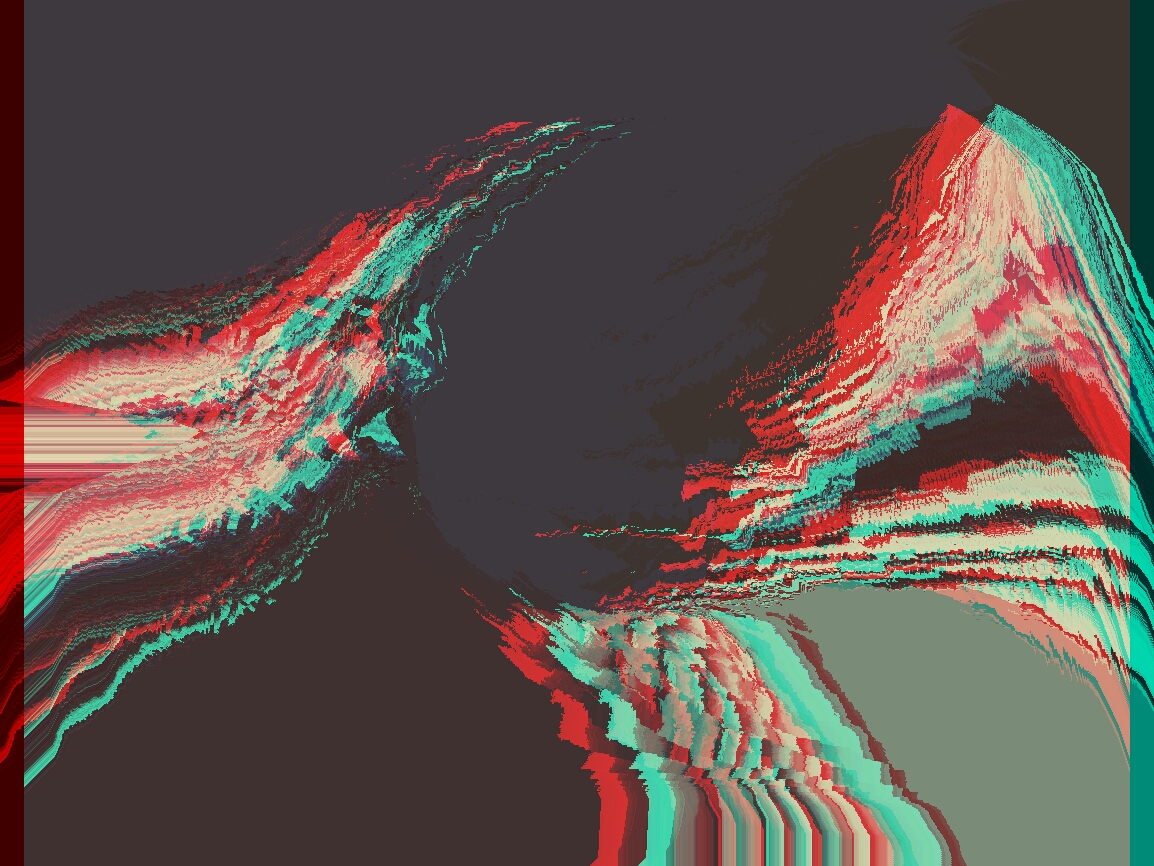This rectangular, computer-generated piece of art showcases a captivating interplay of swirled colors against a dark, almost gray-black backdrop. The image features four distinct sections of color that streak dynamically towards the center, creating a sense of fast movement. From the left emerges a swoosh of vibrant red, turquoise, and white, while from the bottom, a similar burst of colors surges upward. The right side reveals two additional swirls, one after another, blending red, a minty turquoise, white, and hints of pink, further enhancing the visual rhythm. 

The painting evokes the imagery of modernistic waves, with the upper left section resembling a wave cresting and another wave forming on the far right, separated by a central valley. The brushstrokes are fluid and almost blurry, conveying rapid motion. An additional black patch resides in the bottom left corner, contrasting with a smaller but significant olive green area in the bottom right. These elements coalesce into a vivid and dynamic piece that immerses the viewer in an abstract, ocean-like realm defined by its energetic swirls and striking color palette.